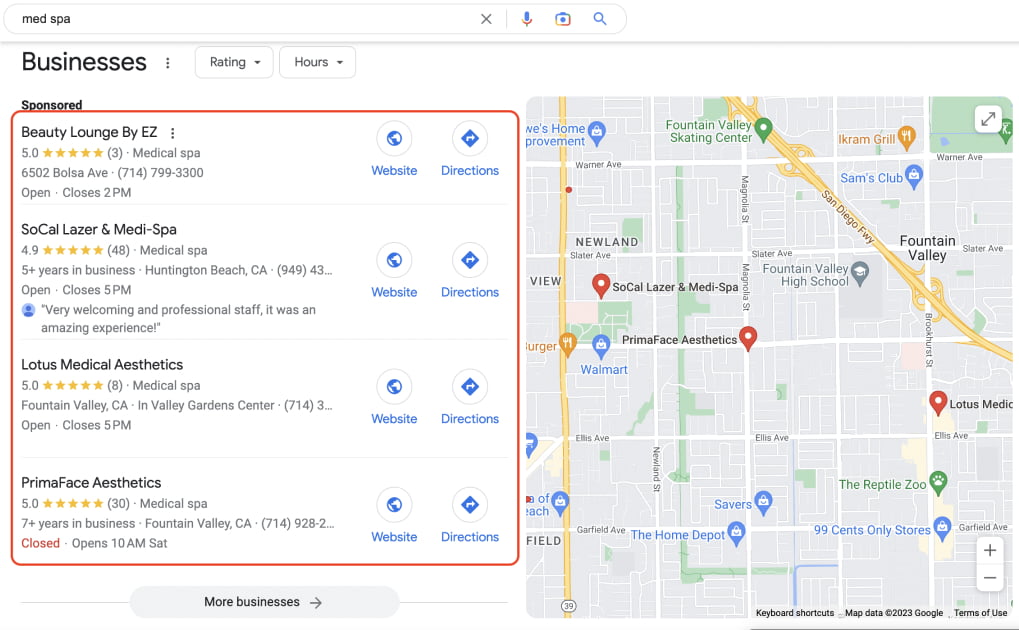A Google Maps interface is displayed, with a search bar at the top containing the query "MedSpa." Just below the search bar, there are categories labeled "Businesses," "Rating and Hours," and "Sponsored." The search results are highlighted within a red box.

1. **Beauty Lounge by EZ**:
   - **Rating**: 5 stars
   - **Reviews**: 3
   - **Type**: Medical Spa
   - **Address**: 6502 Boise Avenue
   - **Phone**: 614-799-3300

2. **SoCal Laser and MedSpa**:
   - **Rating**: 4.9 stars
   - **Reviews**: 48
   - **Type**: Medical Spa
   - **Years in Business**: Over 5 years
   - **Location**: Huntington Beach, CA
   - **Phone**: 949-43…
   - **Hours**: Open, closes at 5 PM
   - There is a generic person icon with a comment stating, "Very Welcoming and Professional Staff, it was an amazing experience."

3. **Lotus Medical Aesthetics**:
   - **Rating**: 5.0 stars
   - **Reviews**: 8
   - **Type**: Medical Spa
   - **Location**: Fountain Valley, CA (in Valley Garden Center)
   - **Phone**: 714-3…
   - **Hours**: Open, closes at 5 PM

This detailed caption thoroughly describes the Google Maps search results for MedSpas, including ratings, reviews, addresses, contact information, and user comments.